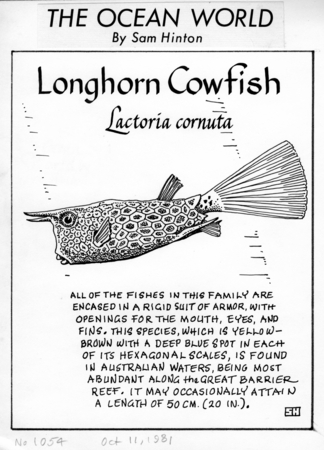The image depicts a black and white illustration, most likely the front cover of a book or a magazine, titled "The Ocean World by Sam Hinton." The background is light gray or white with bold black text. At the top, centrally positioned, is the title "THE OCEAN WORLD" in capital letters, followed immediately by "by Sam Hinton." Below this, there is a prominent rectangular box with a black border and white interior containing additional details. Inside the box, it reads "Longhorn Cowfish," followed by the scientific name "Lactoria cornuta" in italics. The main feature within the box is a black-and-white drawing of a fish with distinctive two horn-like projections at the top of its head, a flat face, and circular patterns on its body resembling hexagonal scales. Below the fish, there is an informative paragraph that explains: "All of the fishes in this family are encased in a rigid suit of armor with openings for the mouth, eyes, and fins. This species, which is yellow-brown with a deep blue spot in each of its hexagonal scales, is found in Australian waters, being most abundant along the Great Barrier Reef. It may occasionally attain a length of 50 cm (20 inches)." The letters "S.H." appear in the bottom right corner of the text box, and the background behind the fish illustration includes lines that resemble a ruler, indicating the scale of the fish.